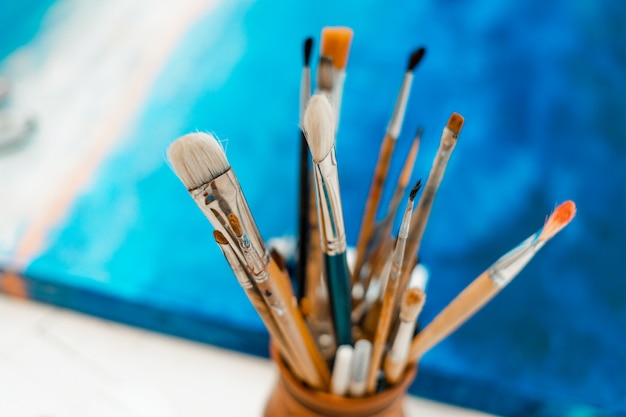This close-up photograph captures an artist's desk, featuring a small brown wooden vase filled with an assortment of various paintbrushes. The paintbrushes, organized bristles-up, display a range of shapes and sizes, with handles in colors including natural wood, black, and a striking teal at the center. The bristles are predominantly white and black, with a few brushes featuring orange-tipped bristles. Each brush is equipped with a metal ferrule that secures the bristles to the handle. The highly detailed paintbrushes in the foreground are in crisp, sharp focus, while the background is intentionally blurred, drawing the eye to the tools of the trade. Behind the vase of brushes, a painted canvas with hues of dark blue, blue, white, and orange sits on a white tabletop, adding a splash of color and context to the workspace.